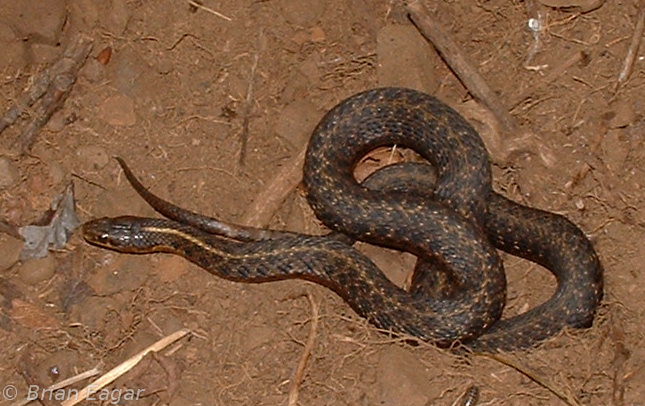This photograph, taken by Brian Ager, captures a long, coiled snake resting on the brown, dirt-covered ground, amidst an area that appears to be near an uprooted tree or a hole. The ground is littered with dead vegetation and roots, indicating a natural and undisturbed setting. The snake, with its dark brown body adorned with faint yellowish lines and varying shades of brown, black, and yellow, lies unaggressively. While the snake lacks the flat head typical of a viper, making it uncertain if it is poisonous, there is a small, half-inch piece that resembles the end of a rattler's rattle visible at the bottom of the photograph, though it is not connected to the snake. The use of flash photography suggests this image was taken at night, as it captures the snake and the surrounding details brightly. The overall scene is devoid of sunlight and human presence, emphasizing the solitary nature of the snake in its natural habitat.